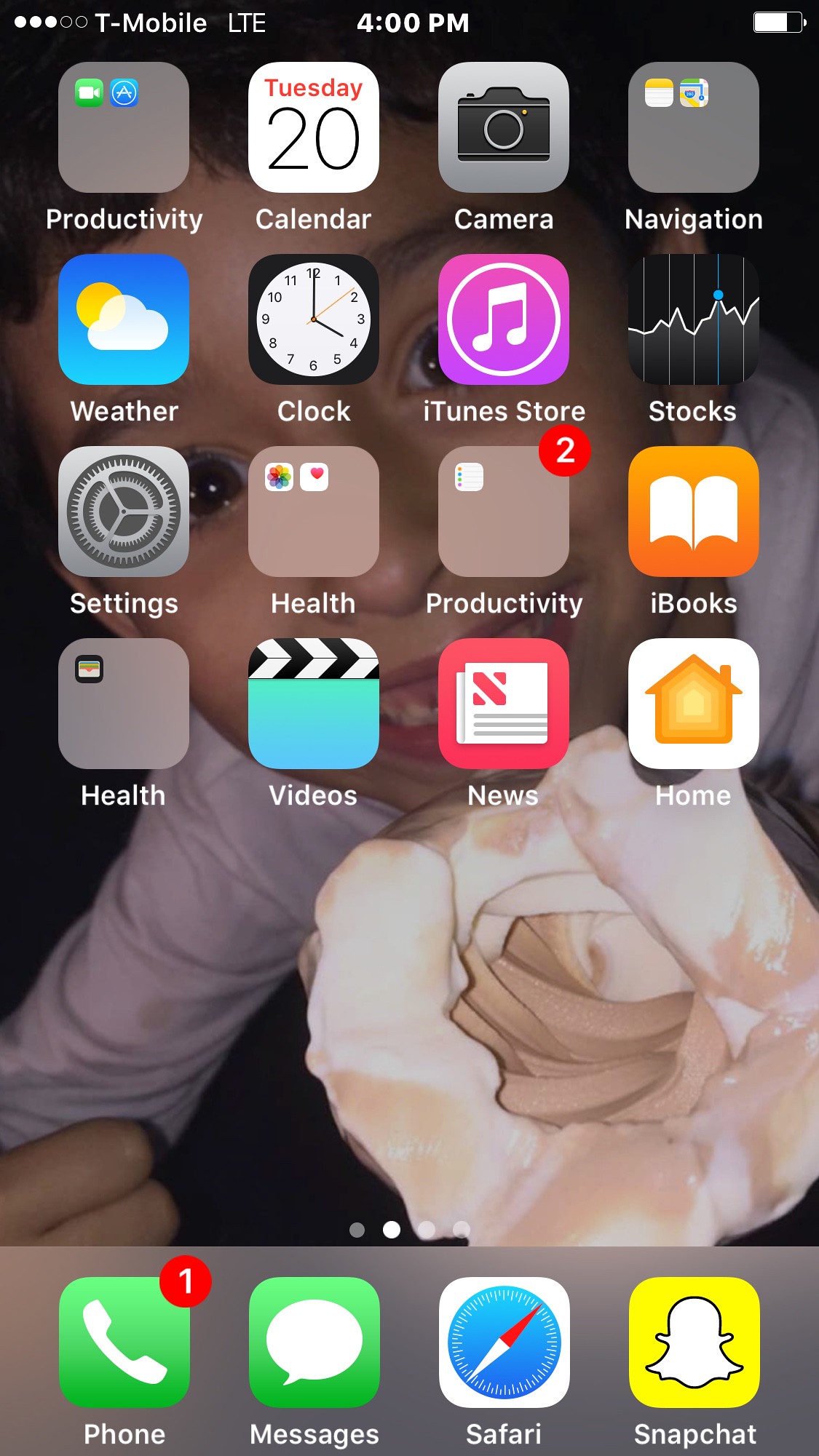This is an image of a cell phone screen displaying a variety of apps against a white home screen background. The phone, a T-Mobile device, shows its signal strength with three out of five dots filled and indicates it is connected to LTE. At the top of the screen, it’s 4:00 PM on Tuesday the 20th, and the battery is approximately 75-80% charged. 

The phone screen displays sixteen apps organized into folders and standalone icons. The visible apps and folders include:
- **Phone**: Indicating a missed call
- **Messages**
- **Safari**
- **Snapchat**
- **Productivity**
- **Calendar** with today's date showing
- **Camera**
- **Navigation** featuring Notes and Maps
- **Weather**
- **Clock**
- **iTunes Store**
- **Stocks**
- **Settings**
- **Health**
- **Gallery**
- **Another Productivity folder** with a single app
- **iBooks**
- **Wallet**, integrated within Health
- **Videos**
- **News**
- **Home**

Underneath these app icons, the dock at the bottom shows frequently used apps, reinforcing the organization's conscious layout for quick and easy accessibility.